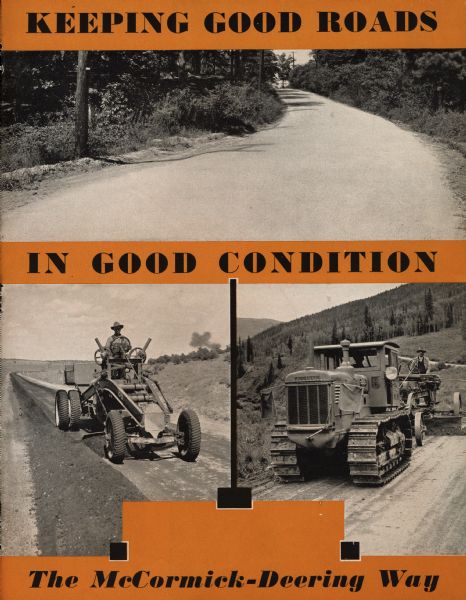This vintage advertisement poster features a striking design with three main sections, each emphasizing the theme of road maintenance and equipment from the past. The top section has a bold orange background adorned with black, capitalized text that reads, "Keeping Good Roads." Below this, a black and white image of a well-paved road is flanked by grass and trees, symbolizing the ideal of pristine road conditions. The middle section, also with an orange background and capitalized black text, states, "In Good Condition." The bottom section showcases two black and white images, split in half. On the left is a detailed depiction of a classic, open-cab farm tractor with a driver operating it, visibly moving soil beneath. On the right is a larger tractor with tank treads and a front scoop blade, accompanied by two men—one standing by the blade and another walking beside the vehicle. Underneath these images, another orange bar with black text proclaims the company's name, "The McCormick Deering Way," emphasizing their role as equipment manufacturers dedicated to maintaining road quality.